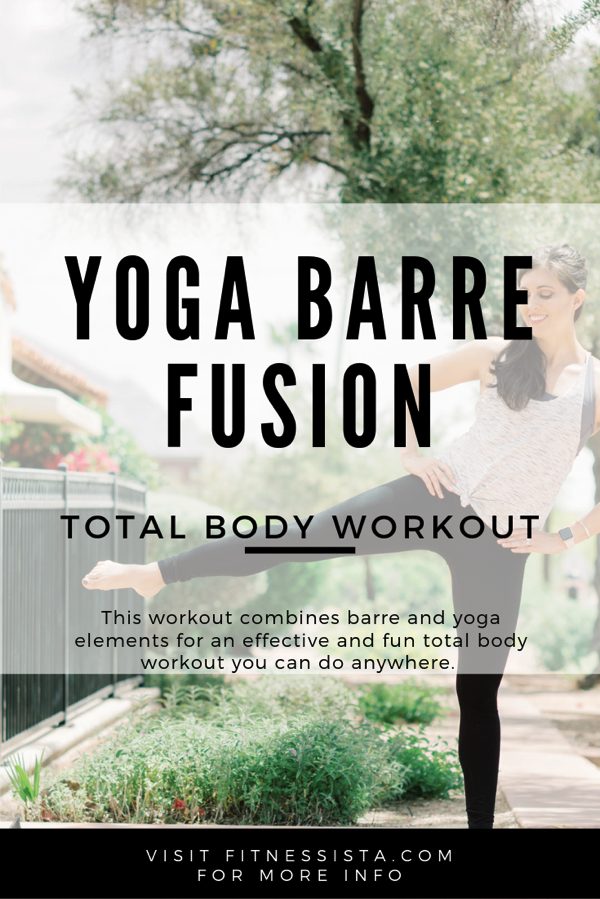The image is a rectangular promotional flyer, approximately six inches tall and four inches wide. At the bottom of the flyer, there's a black footer occupying about half an inch in height, stretching across from the lower left to the right corners. Centrally positioned within the black footer, in two rows of white lettering, is the text "visit fitnessista.com" for more information.

Above the footer, the primary background image features a Caucasian woman on the right side performing a yoga pose. She stands on her left leg with her right leg extended sideways at the hip, placing her hands on her hips. She has brown hair tied back into a ponytail that drapes over her shoulder. Her attire consists of a light-colored tank top and black stretch pants. The setting is an outdoor sidewalk scene, with a tree directly behind her and a metal fence with foliage to the left.

Overlaying the center of the image is a transparent white banner with bold black text at the top, stating "Yoga Barre Fusion: Total Body Workout." Below this header, it explains, "This workout combines barre and yoga elements for an effective and fun total body workout you can do anywhere."